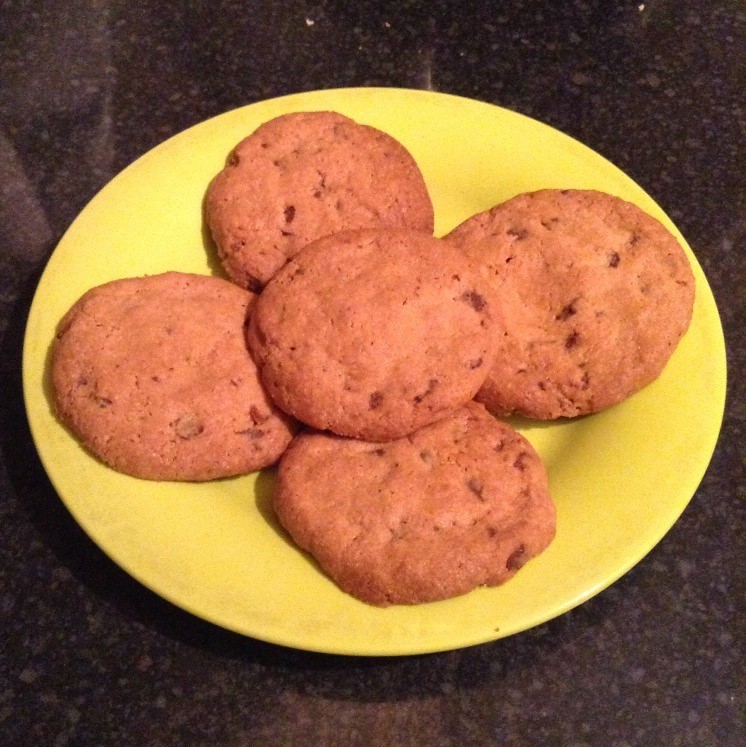This image features a detailed close-up of a yellow, undecorated plate holding five homemade cookies, arranged to resemble a flower. The plate, a medium lemon yellow, sits on a polished black granite countertop adorned with lighter brown splotches. Four golden brown cookies form the bottom layer, each sprinkled with darker specks that could be chocolate chips or raisins, and display varying degrees of crispiness and size. At the center, on top of these four, rests a single cookie, forming the second layer. The cookies collectively create an aesthetically pleasing arrangement that draws the viewer's eye to the center. There's also a small dark speck on the lower edge of the plate, likely a stray crumb.